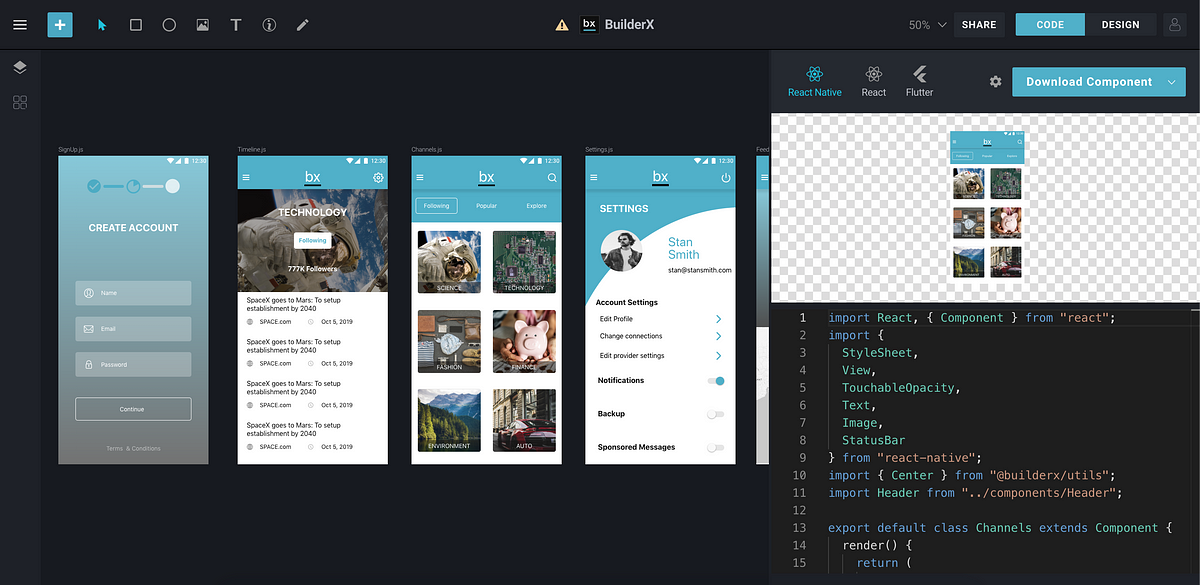On the webpage with a solid black background, the top left corner features a set of three horizontal white lines, each approximately half an inch long, stacked vertically. Directly below, there's a diamond-shaped element with a grey lower half. Adjacent to it are three black circles, each encased in a grey border, forming a square arrangement.

At the top center, a blue square with a white plus sign and an upward-pointing white arrow draw attention. This is followed by a sequence of UI elements: a black square with a grey border, another black circle with a grey border, an icon representing a picture, a large grey "T", a circle with a grey eye inside it, and a grey pencil icon. Next, there is a profile icon, and tabs labeled "Design," "Code," and "Share" in white font on black, blue, and black backgrounds respectively. Nearby, a display shows "50%" moving leftwards.

In the center, a yellow triangle containing a black exclamation mark is prominently displayed, next to a black square with "BX" underlined in blue and the text "Builder X" beside it. Below this, four phone outlines depict sequential steps for accessing settings, arranged horizontally from left to right.

The right third of the screen features icons for React Native, React, and Flutter, as well as a settings icon. A blue rectangle with the white text "Download Component" is positioned below these icons, followed by a checkerboard pattern in white and black. The central portion includes another blue rectangle and three vertically aligned pictures flanked by two horizontally aligned images. The bottom section displays coding lines numbered 1 through 15.